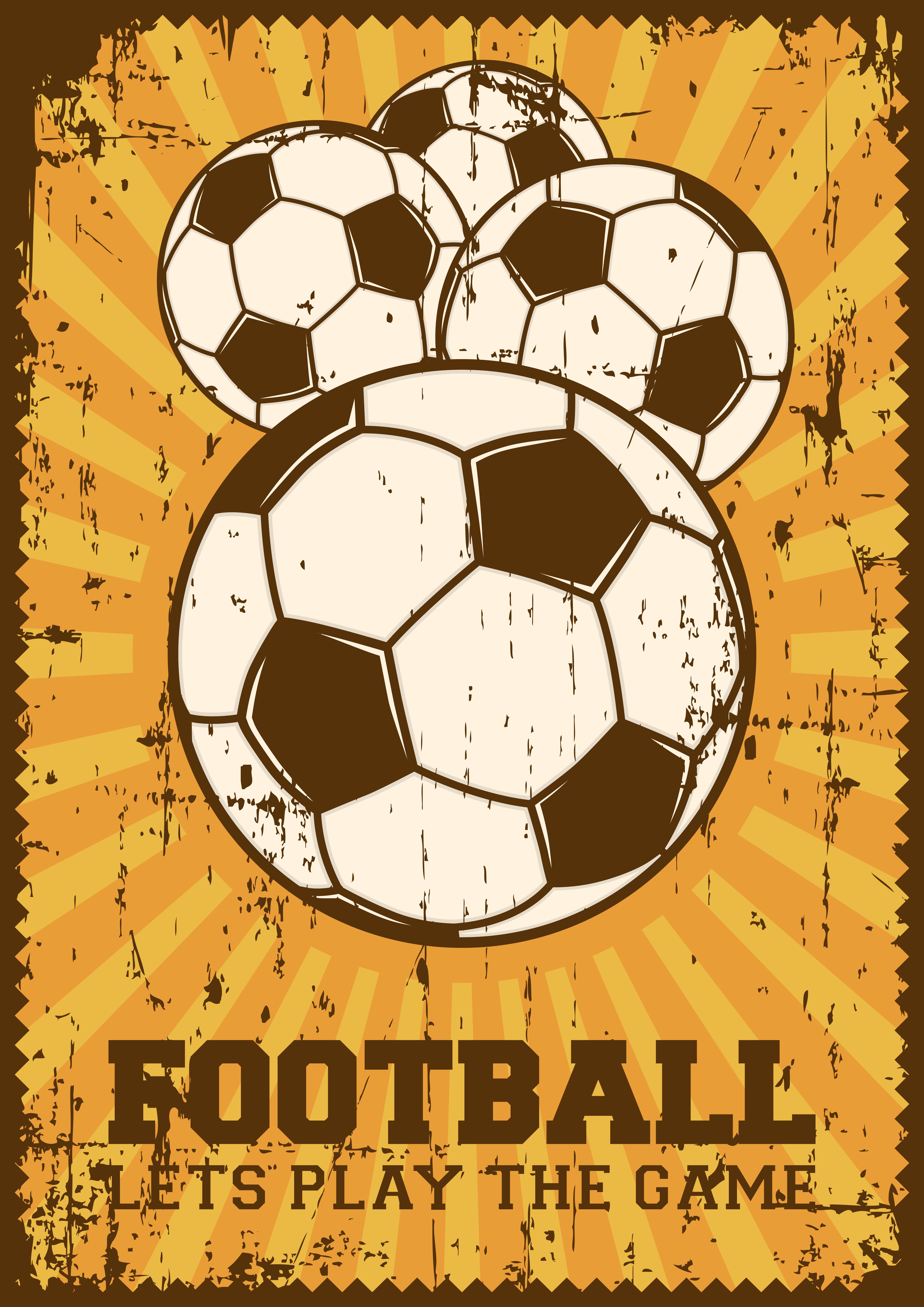The image is a vertical rectangular poster featuring a central composition of four European footballs, or soccer balls, characterized by their white backgrounds with brown pentagons. These balls are arranged in front of a radiant sun, with rays streaming out to the border in alternating shades of peach and light mustard yellow. The entire poster is framed by a dark brown border. At the bottom of the poster, there is a text in brown font that reads, "Football, let's play the game."